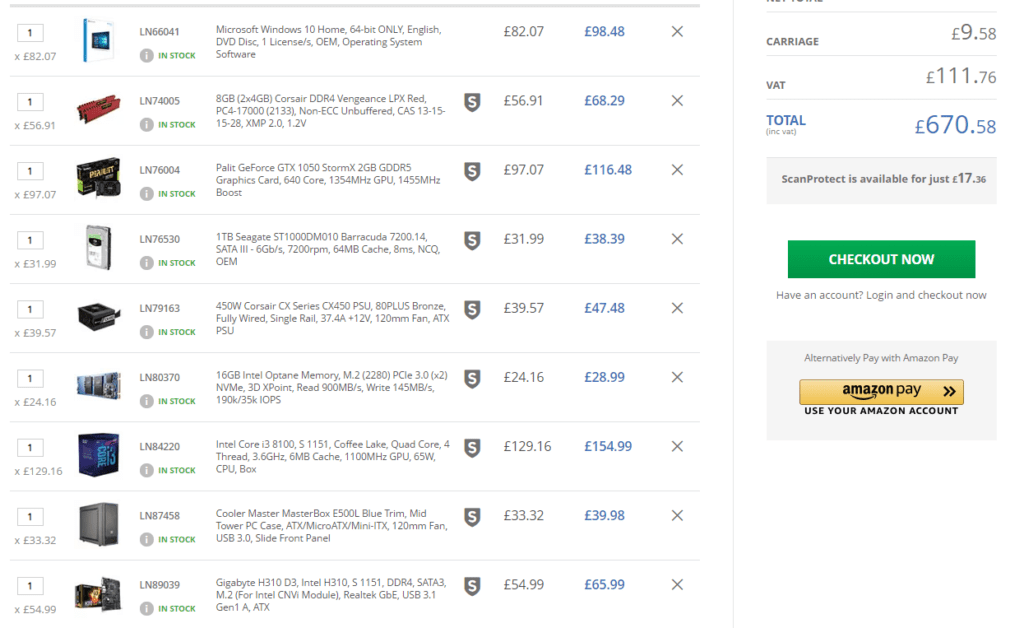This image depicts a shopping cart screen displaying various computer components, organized into a detailed tabular format. The screen contains nine entries, each representing a different item available for purchase. Starting from the left, the first column shows the quantity selected and the corresponding total price for each component.

Adjacent to this, each item is visually represented by a thumbnail image in the second column. The third column contains the item number and the stock status, with "In Stock" entries prominently highlighted in bright green to indicate availability.

The fourth column provides a comprehensive description of each computer component, followed by the fifth column which lists the unit price. An intriguing detail is found in the sixth column, where figures appear in bold blue. Although it's not clarified, this might represent a price inclusive of tax, potentially the VAT charge, as suggested by the summary section on the right side of the screen.

Taking up roughly the rightmost 25% of the screen, this summary section includes specifics like the carriage fee and VAT fee, supporting the hypothesis about the extra costs accounted for in the bold blue figures. 

For user convenience, there are two prominent buttons for completing the purchase: one for standard checkout and another for Amazon Pay.

Intriguingly, between the description and unit price columns of the bottom eight entries, there's a shield icon with an 'S' in white, set against a gray background. However, its purpose remains unclear due to the absence of an explanatory legend.